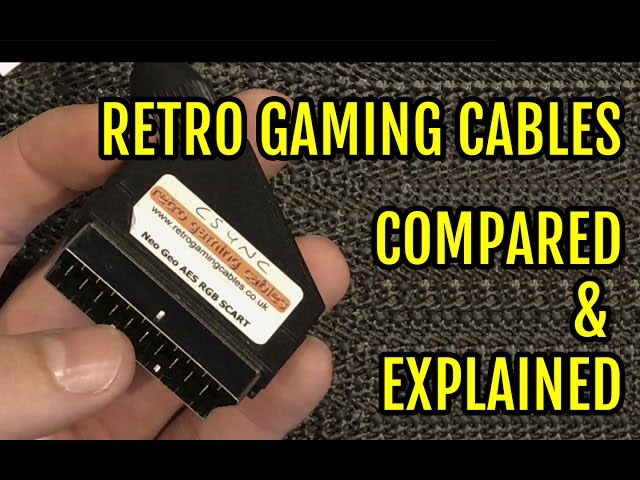This wide, horizontal image features a detailed, zoomed-in view of a gaming card, predominantly held by a hand whose five fingers are visible. The gaming card, black with a gradient darker black towards the bottom, displays the text "CSYNC" at the top, followed by "Retro Gaming Cables" against an orange background, the URL "www.retrogamingcables.co.uk," and "NeoGeoAESRGBSCART" at the bottom. On the right side, large yellow text reads "Retro Gaming Cables Compared and Explained," set against a dark gray, carpet-like background, with black borders on the top and bottom, suggesting the image might serve as an introduction to a video about retro gaming cables.